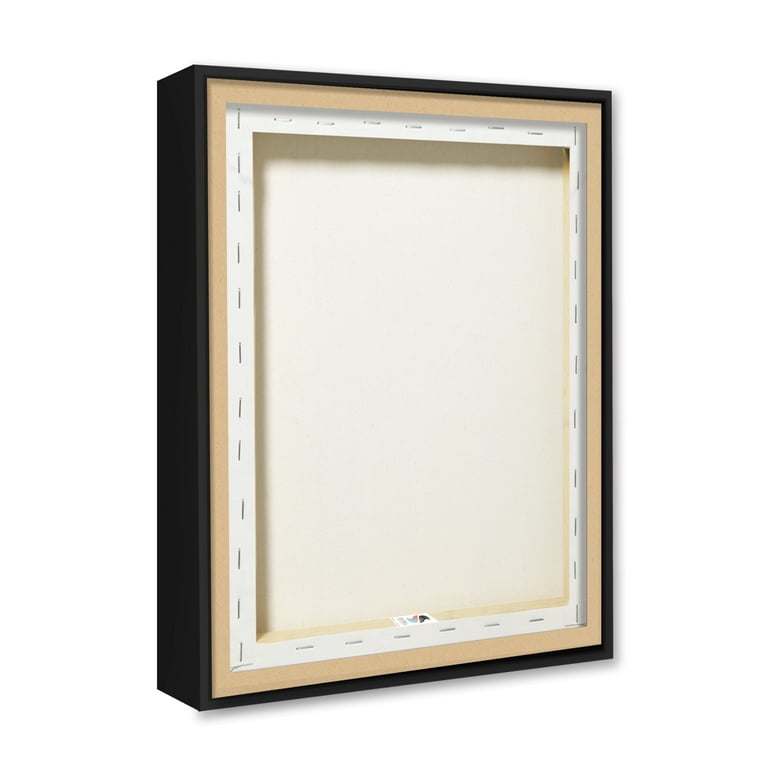This image captures the backside of a black frame that is approximately three to four inches thick. The interior reveals a wooden structure supporting a cream-colored canvas, which has been securely stapled along the edges. The staples are methodically placed across all four corners, running the entire length and breadth of the canvas. A notable detail includes a small label at the bottom center of the wooden piece, featuring a swirl design in blue and pink, accompanied by a smaller black swirl. This label appears to be partially unreadable, noting what seems to be the letters "IVA" or something similar. The overall image is minimalistic, displaying only the back of the frame and its components, as well as an impression of a shadow underneath and to the right, possibly indicating that the photo serves a promotional or illustrative purpose.